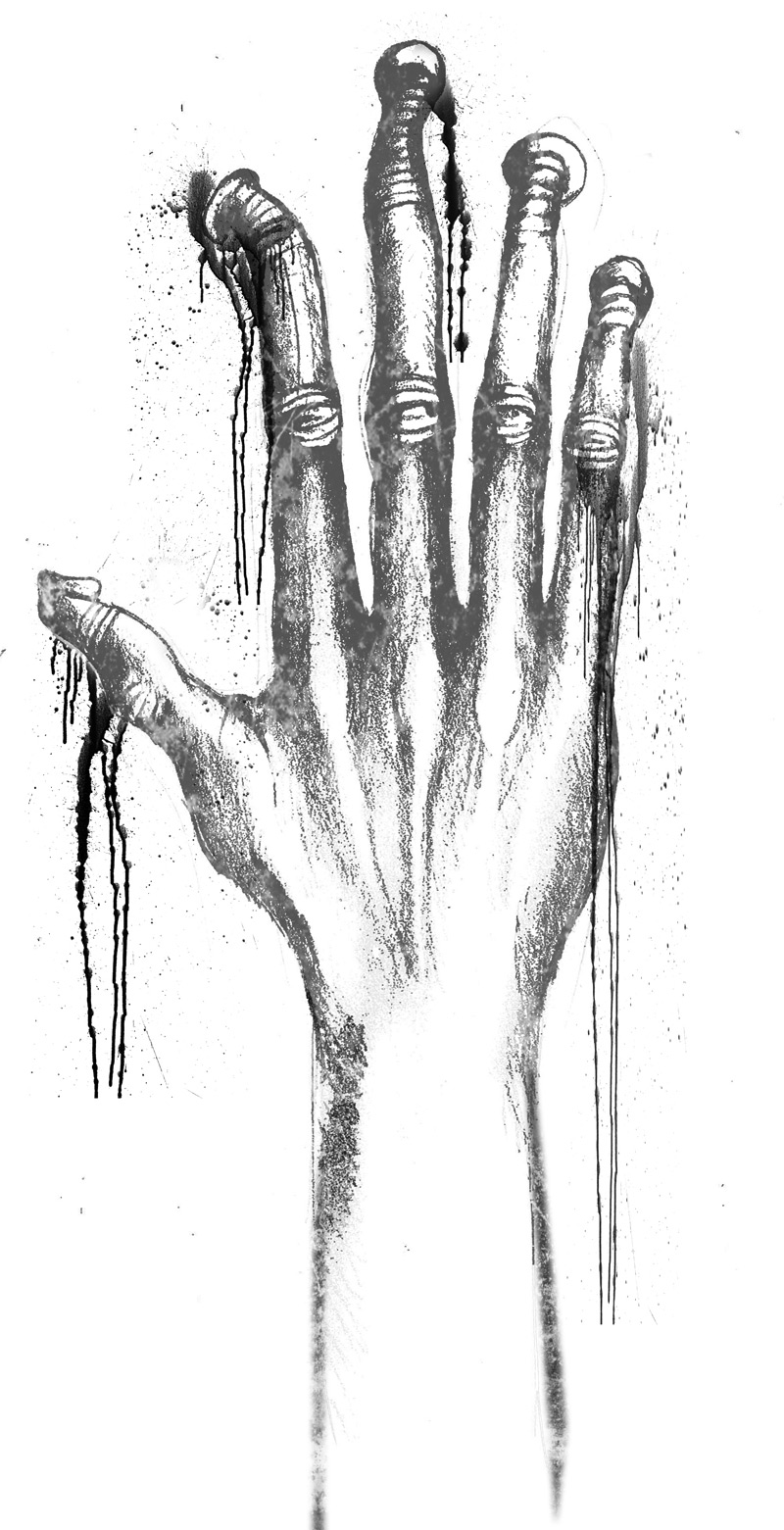This black and white drawing, likely created with pen and ink, showcases a detailed depiction of a right hand and part of the forearm extending upward from the bottom of the image. The hand is stretched out, with all five fingers splayed and touching an indistinct surface that appears to press against the fingers. Each fingertip is adorned with a small piece of cloth or bandage, from which slender black strings or strands hang down conspicuously. Some of these strands, particularly from the thumb, index, middle, and pinky fingers, seem to be longer and darker, suggesting blood dripping from the contact points with the surface.

The drawing extends roughly four to five inches past the wrist, emphasizing not only the fingertips but also the forearm. The hand is delineated with bold shading and significant black markings, particularly accentuating the knuckles and the varied textures across the hand. This stark contrast in shading gives the drawing a vivid and dramatic appearance, while the white background provides no additional context, focusing the viewer’s attention entirely on the intricacies and starkness of the hand's portrayal.